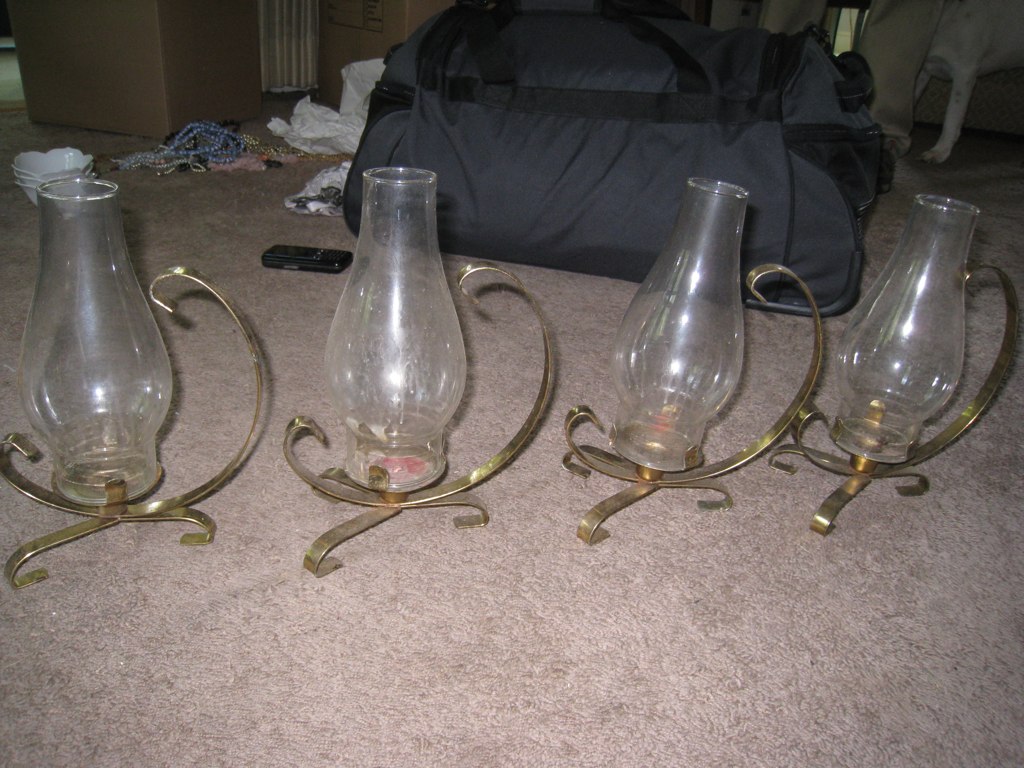This vibrant color photograph captures an indoor scene illuminated primarily by the camera's flash, emphasizing four similar cylindrical lanterns on a beige, low-pile carpet. Each lantern consists of a clear glass holder with a bulbous shape—wider at the base and narrowing towards the top—set in a simple curved gold/brass metal frame with handles on both sides. Scattered around in the cluttered background on the pinkish-gray rug are various items, including a cell phone lying to the left, a large black duffel bag, clothing, necklaces, cardboard boxes, and a stack of three white scalloped bowls. Additionally, part of a dog nestled into the curtains can be seen, hinting at a cozy, albeit messy, domestic setting.